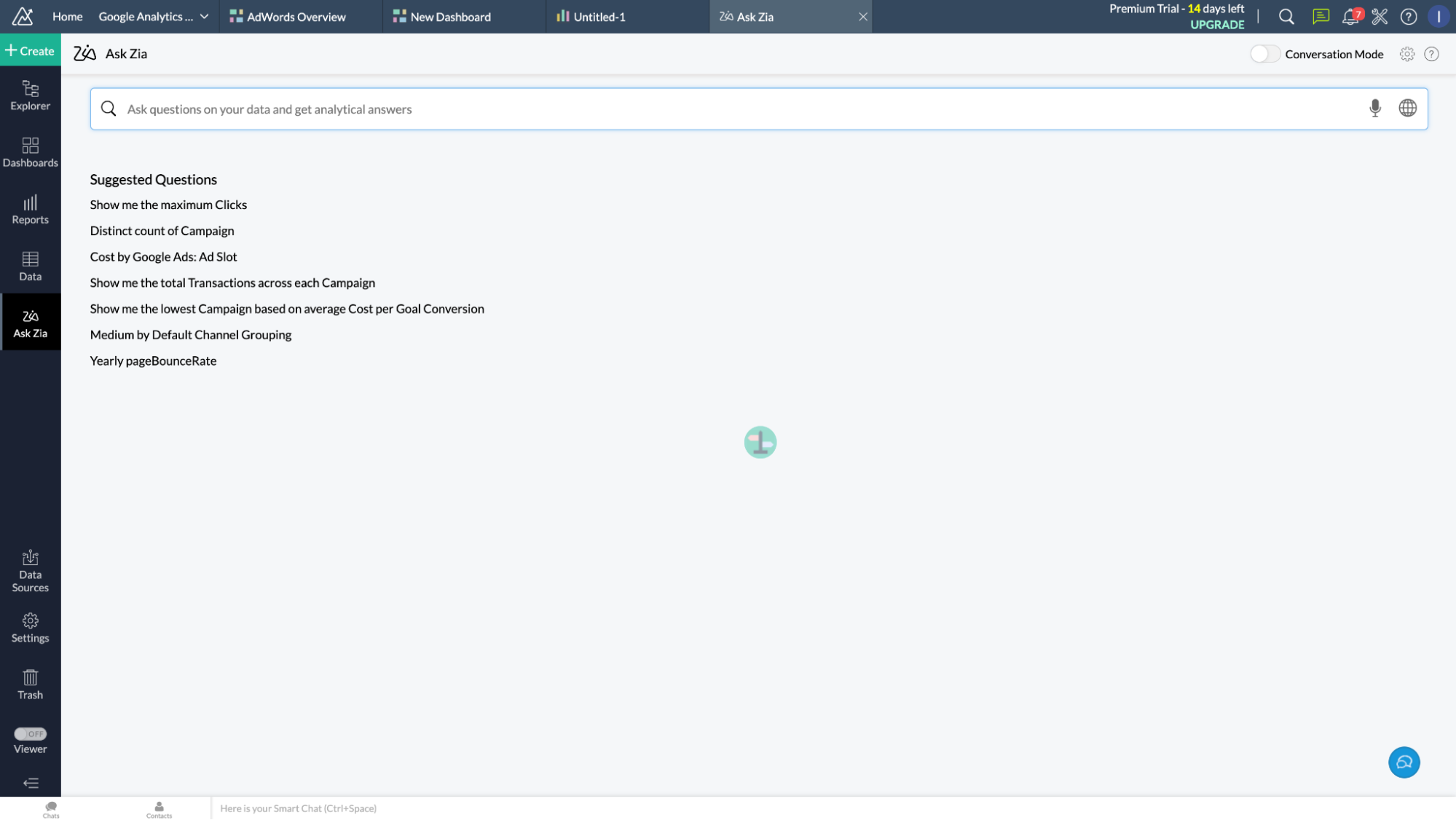### Detailed Screenshot Description: Google Analytics Dashboard Interface

The screenshot captures a Google Analytics dashboard interface in landscape orientation displayed on a laptop screen. 

**Header Row:**
The top row of the interface features a dark gray background. The following tabs are aligned from left to right:
- **Home**
- **Google Analytics**
- **AdWords Overview**
- **New Dashboard**
- **Untitled 1**
- **Ask Zia** (highlighted tab indicating it is currently active)

Next to the tabs:
- **Premium Trial, 14 days left** with an option to upgrade in light green.
- A **search bar** for easy navigation.
- **Seven notifications** indicated by an icon with a number.
- An **eye icon circled at the upper right-hand corner** possibly for viewing settings.

**Sidebar (Left Column):**
The sidebar on the left contains navigational elements as follows:
- **Plus Create** button in a green box for creating new reports or dashboards.
- Categories listed include:
  - **Explorer**
  - **Dashboards**
  - **Reports**
  - **Data**
  - **Ask Zia** (highlighted, likely selected)
  - **Data Sources**
  - **Settings**
  - **Trash**
  - **Viewers**

**Main Content (Right Column):**
At the top of the main content area is a header labeled **Ask Zia** with **Conversation Mode toggled off** on the right side.
Directly below, a white search box with the prompt **"Ask Questions on Your Data and Get Analytical Answers"** appears. At the end of this search bar, there is a microphone icon, indicating voice input options.

**Suggested Questions Section:**
The following suggested analytical queries are displayed in bold under the search bar:
- Show Me the Maximum Clicks
- Distinct Count of Campaign
- Cost by Google Ads
- Ad Slot
- Show Me the Total Transactions Across Each Campaign
- Show Me the Lowest Campaign Based on Average Cost per Goal Conversion
- Medium by Default Channel Grouping
- Yearly Page Bounce Rate

**Visual Element:**
In the center of this section, a small green circle featuring an icon that resembles either a building or a flagpole with clouds, yellow and white, serves as a visual element, adding a touch of graphical interest to the interface.

**Lower Right Corner:**
A blue conversation icon is located at the bottom right-hand corner, likely for accessing help or support features.

This detailed description provides a thorough understanding of the Google Analytics dashboard interface and its various components as depicted in the screenshot.